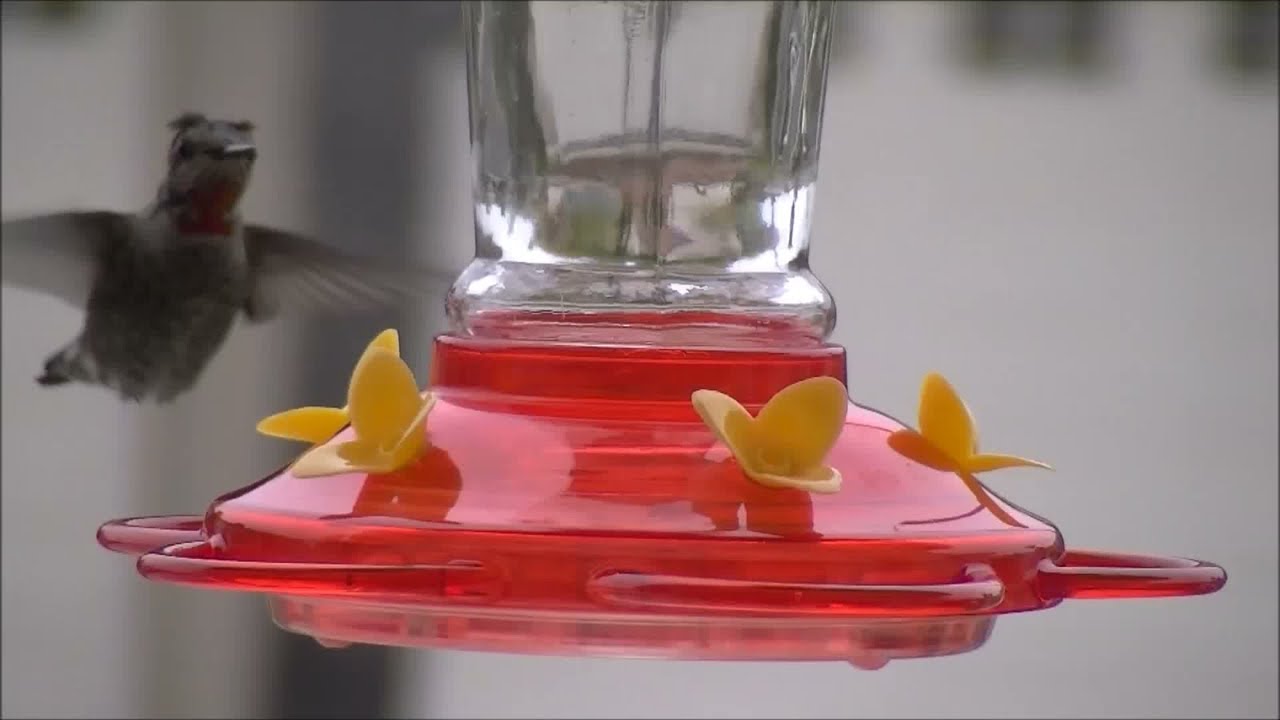An outdoor close-up photo captures a hummingbird at a feeder. The feeder features a translucent tall glass cylinder for nectar, topped with a red, slightly transparent plastic base. Attached to the base are yellow plastic flowers, each with three petals and a small central hole for feeding. Surrounding the base are four perching handles: two on the sides, and two facing forward. A dark brown to black hummingbird perches on the left handle, its long beak inserted into one of the flower openings. The bird's claws visibly grip the handle, and one eye appears open. The background of the image is completely blurred.